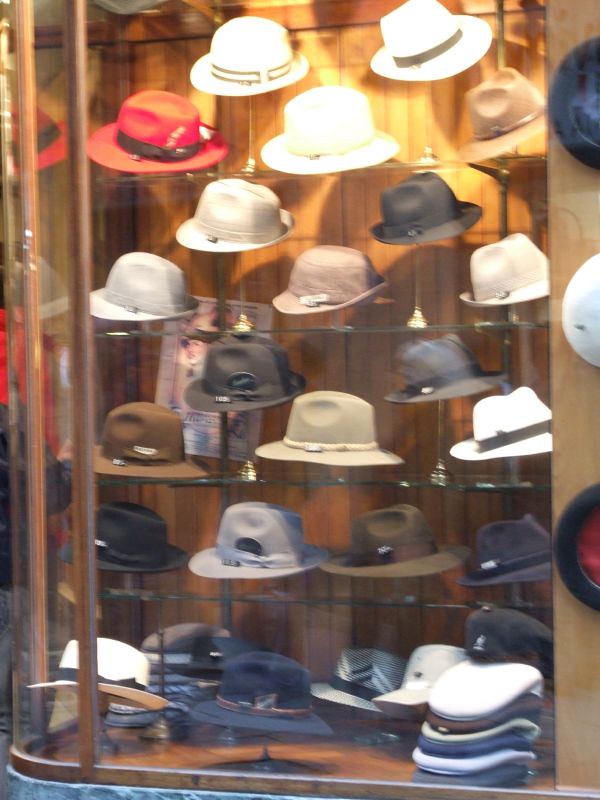The photograph showcases a detailed display of a varied collection of wide-brimmed hats arranged in a glass case with a wooden backdrop. The hats are mounted on black wire stands and organized in horizontal rows, creating a staggered effect towards the top. The collection includes an array of styles: classic fedoras, military-style hats in olive green, and wide-brimmed hats reminiscent of Australian outback style. Prominently featured at the top left is a striking red hat with a black ribbon. The hats come in multiple colors, including white, brown, tan, gray, blue, and black, each adorned with ribbons or bands. The bottom section of the display case hosts a more casual assortment, with a pile of sports car caps and flat caps situated on a wooden floor. The overall scene encapsulates the diversity and elegance of hat styles, set against the warm, wooden paneling background and accented by circular windows and a crooked picture frame in the middle of the image.